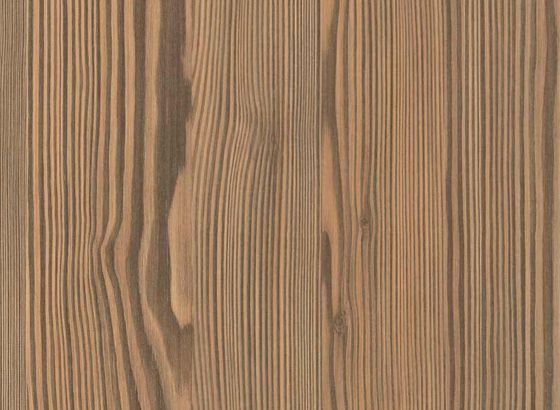The photograph is a detailed close-up of a wooden plank surface, showcasing its intricate grain patterns and varying line densities. The wood, in shades of dark brown to light tan, features vertical age lines that run parallel to each other with subtle curves. On the left side, the lines are densely packed together, then gradually spread apart towards the center, where they contract again. As the lines move towards the right edge, they first normalize and finally become widely spaced once more. The entire surface gives the impression of being composed of different segments, with the detailed wood texture creating a visually interesting pattern that is consistent throughout the image. The background hues range from dark brown to a pinkish medium tan, adding to the rich, natural appearance of the wood.